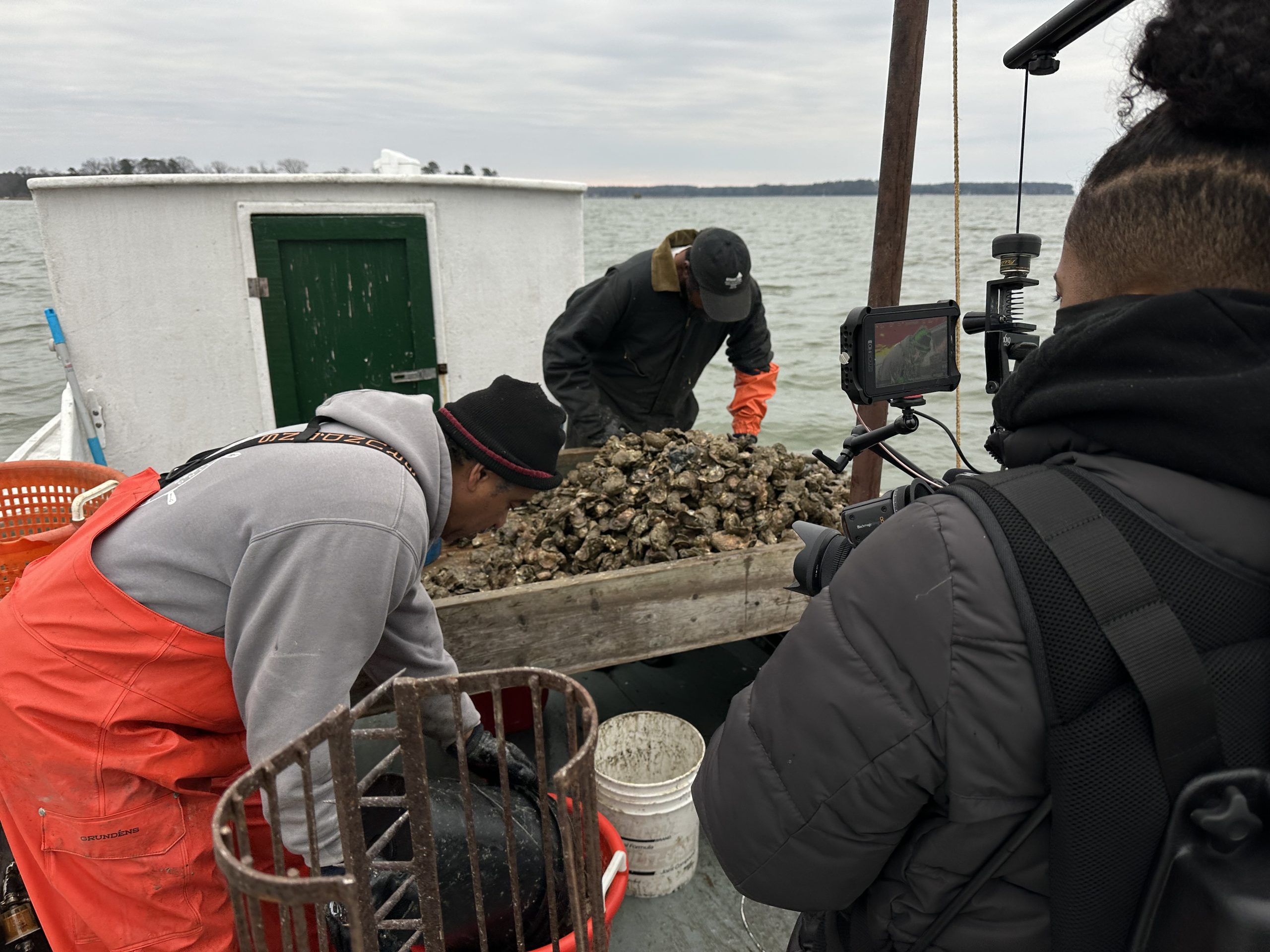The photograph captures a scene aboard a bustling fishing vessel on a gray, overcast day with turbulent, greenish waters. Three fishermen are diligently at work on the deck, which features lobster traps and empty buckets. The fisherman closest to the camera, possibly a female, is dressed in distinctive orange rubber overalls, a gray sweatshirt, and a black knit cap. The second fisherman, farther back and equipped with a black nylon parka, appears to be using a depth finder attached to a pole. The third fisherman, bent over and dressed in black, meticulously sorts through a full tray of shellfish or rocks, suggesting a day of shellfishing or dredging. In the background, the white cabin of the boat with a black door stands out against the cloudy sky. The scene vividly captures the hardworking nature of the fishermen amidst the challenging, stormy sea conditions.